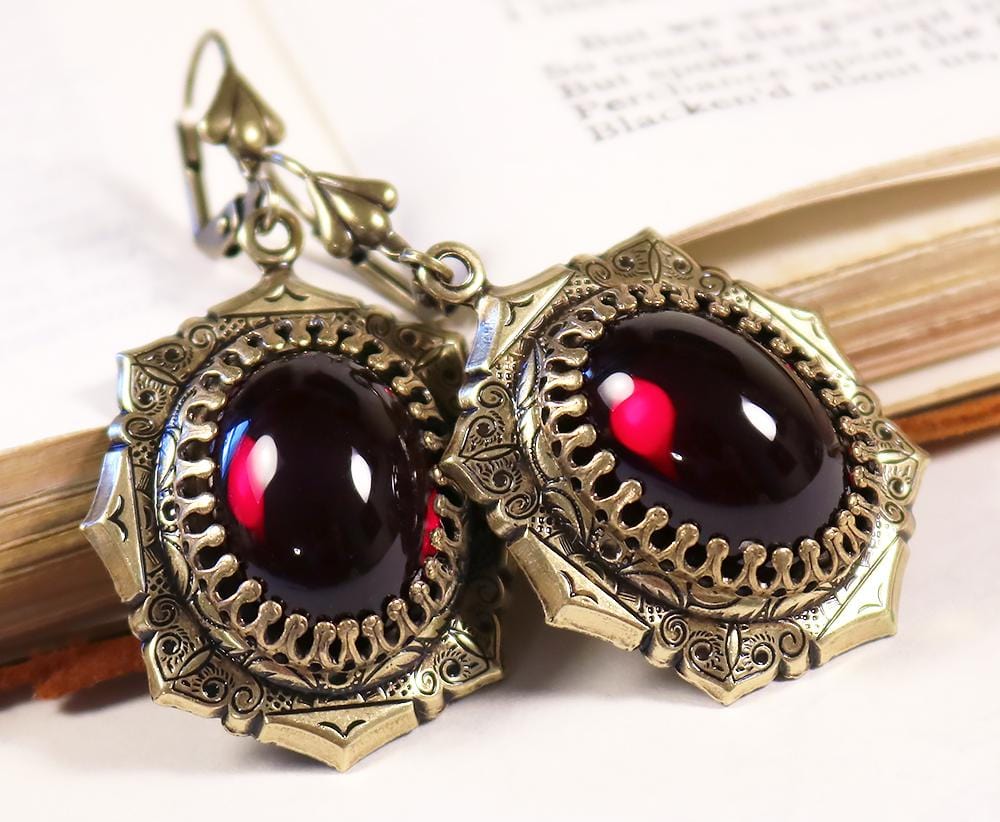In this detailed image, there are two striking earrings positioned against an open, slightly aged book with indistinct text on its yellowed pages. The earrings, designed for pierced ears, feature a gold-ish, octagon-shaped setting that houses an oval black stone with subtle red highlights. This central gem is encased in a crown-like decoration and has additional carved swirls and detailing around the edges, giving it a somewhat bulky appearance. The gold metal setting seems slightly stamped and ornate, extending into hoops at the back for ear-dangling. The book in the background is open and faded, with parts of its text visible but unreadable. Everything rests on a white surface beneath the book and the earrings.